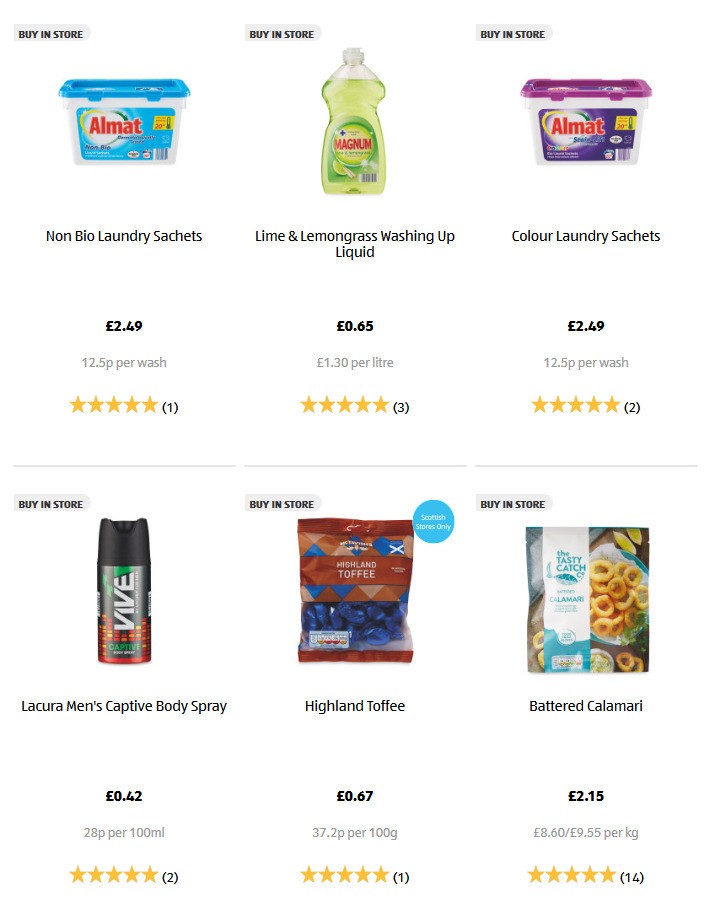This screenshot captures a page from an unspecified shopping app, showcasing six diverse products. Each product is accompanied by a price listed in either euros or pounds, as well as a star rating out of five stars. The items on display include: Non-Bio Laundry Sachets, Lime and Lemongrass Dishwashing Liquid, Colored Laundry Sheets, Lacura Men's Captive Body Spray, Highland Toffee, and Battered Calamari. Each product is clearly positioned to inform the customer of its cost and user rating, providing a comprehensive snapshot of the available options.